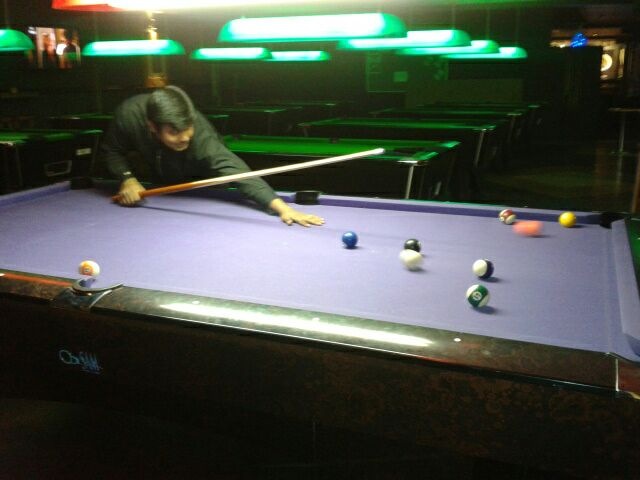The photograph captures a young man intensely focused on a game of pool in a dimly lit bar or pool hall with low ceilings. He is standing at the corner of a pool table covered in blueish-purple felt, aiming a pool stick with his left hand flat on the table. A solitary orange ball is visibly in motion, suggesting he has just taken a shot. His attire, a black sweater, highlights his composure and dedication to the game. The scene is illuminated by green lights suspended above, casting a greenish glow that accentuates the green felt edges on the numerous pool tables lined up behind him. The background reveals a series of vacant pool tables stretching into the distance, with around eight green lights hanging above them. A TV is mounted in the corner of the room, and neon lights—a blue and a white one—add to the ambiance of the space. Various colorful balls are scattered across the table, emphasizing the ongoing game.